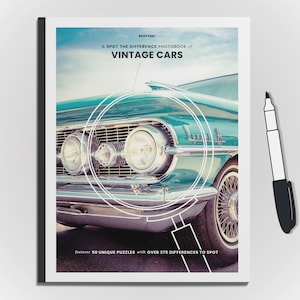The image showcases a gray-background booklet or magazine with a black spine and a white border around the front cover. The cover features a detailed photograph of a restored vintage car, likely a Ford Mustang, in aqua green or turquoise. At the top, the title "Vintage Cars" is written in black font, with some smaller and blurrier black text above it, possibly reading "Spotted: A Spot the Difference Photo Book of Vintage Cars." Centered over the front left headlight is a white outline of a magnifying glass, creating a focal point effect. The vintage car, with round silver headlights, a silver front bumper, black tire with a white sidewall, and silver-spoked steel rims, is set against an asphalt ground with a blue sky and fluffy clouds in the background. Small white text at the bottom of the cover is too blurry to decipher. Adjacent to the booklet, there is a black and white felt tip pen.